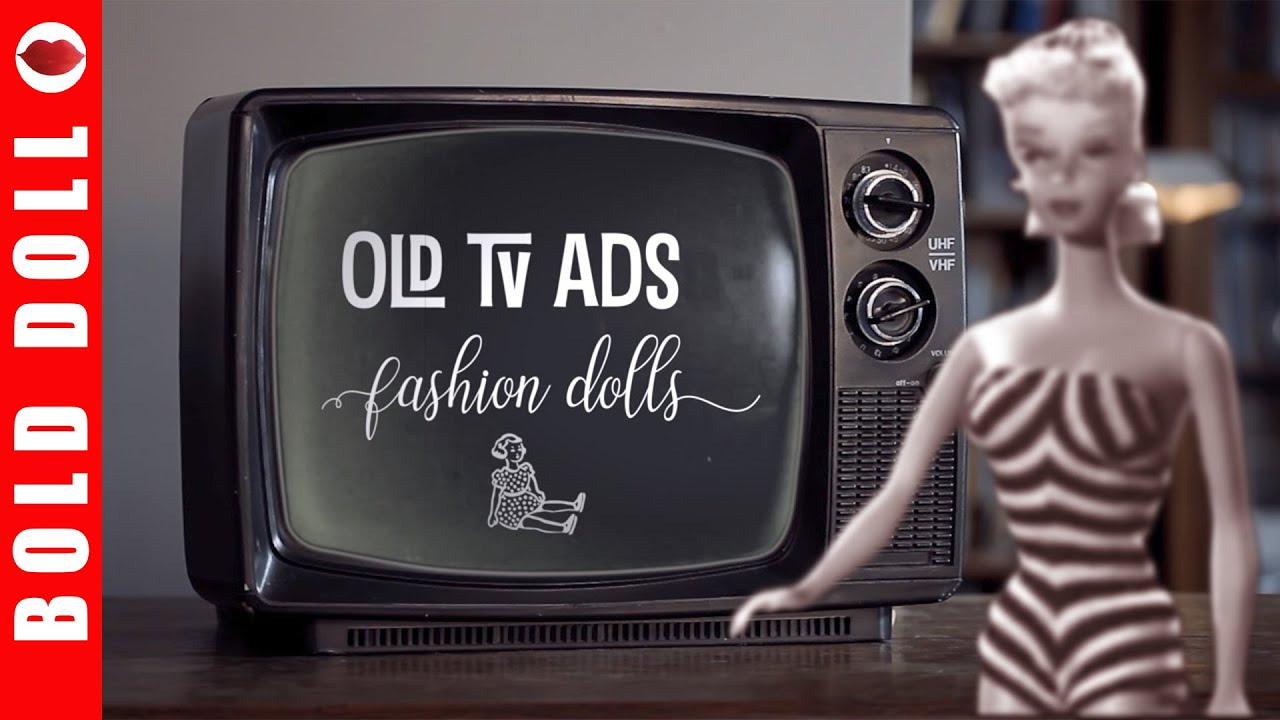The image depicts a vintage black-and-white television displaying an ad titled "Old TV Ads: Fashion Dolls," with the text written in italicized white cursive. Below the text, there's a minimalistic graphic of a doll seated on its butt. The TV, situated centrally in the image, features two dials on the right side, hinting at its analog nature. Positioned in the foreground to the right, slightly blurry and out of focus, is a female doll with light blonde hair, dressed in a black and white striped outfit resembling an old-style swimsuit. On the left side of the picture, a red banner with the product name "Bold Doll" is prominently displayed in a white, capitalized font, accompanied by a graphic of lips at the top.